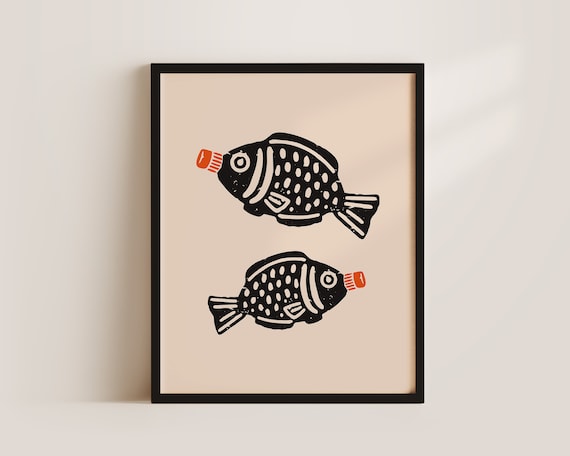In the picture frame, there are two black fish intricately drawn with white eyes, white lines, and white fins. Their tails boast four white stripes each against the black, while the fins and bodies are decorated with white dots and stripes. The unique feature of these fish is their orange-tipped noses, resembling twist-off caps, adding a distinctive characteristic to their appearance. The fish are facing opposite directions—one facing left and the other right—with each facing upward in the design. The background of the artwork is a pristine white, providing a stark contrast to the black fish and their detailed white markings. This is all set within a sleek black frame, which further emphasizes the light, clean aesthetic of the picture against a white wall. The overall composition exudes a modern and minimalist style, highlighted by the symmetry and contrasting colors.